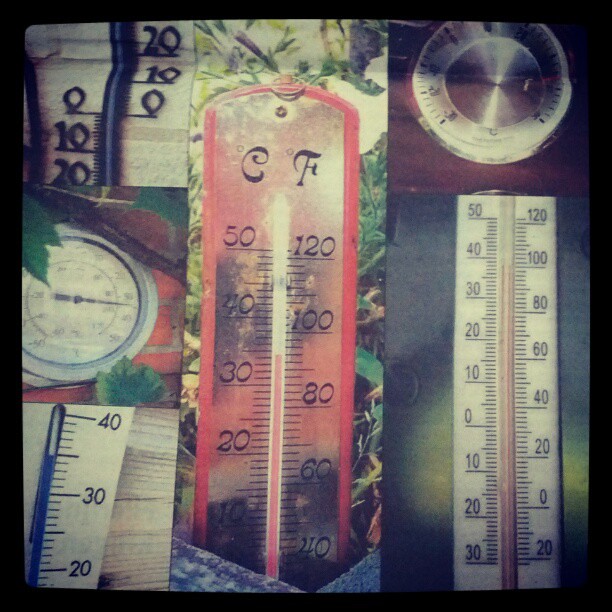The image is a square photograph featuring a printed sheet of paper displaying six different outdoor thermometers, each with unique designs. The photograph itself has a well-defined, thin black border on all sides, which outlines the squared paper and its content.

The sheet of paper, also square, exhibits a slight crease running diagonally from the top left corner to the top right corner, suggesting it had been folded previously. Arranged vertically along the left side of the paper are three different styles of thermometers:

1. At the top left, there is a thermometer mounted on a piece of brown wood. The thermometer features a black center with black numbers on either side, likely for temperature readings.
   
2. Directly below it, a circular thermometer is affixed to a red brick wall. This thermometer has a white face and a black needle, which points towards the temperature scale marked around the edge.

3. Further down, a traditional-style thermometer with a white and black design is noted. It contains black liquid inside a vertical tube, accompanied by black notches and numbers for temperature measurement.

Each thermometer representation on the paper is captured in detailed photographs, showcasing the variety in style and mounting possibilities, offering a comprehensive visual guide for comparing different outdoor thermometers.